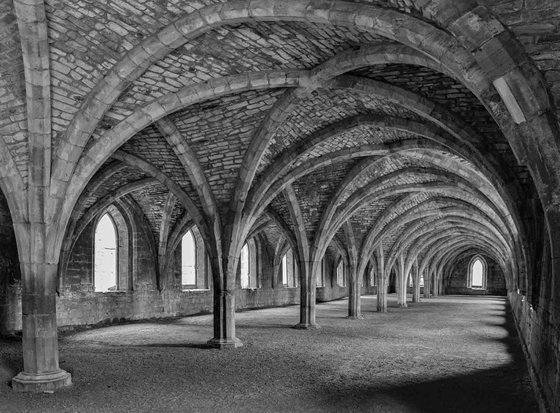This black and white photograph captures the intricate interior of a cathedral or monastery, showcasing a long corridor adorned with tall, stone archways that stretch from floor to ceiling. The archways, resembling the branches of a tree, converge upon central stone pillars placed at regular intervals down the corridor. The stone and brick structure displays a geometric pattern that repeats throughout, contributing to the overall depth and harmony of the scene. Arched windows on the left side of the corridor allow light to penetrate, casting shadows that contrast with the otherwise dim interior, highlighting the detailed masonry work. The smooth, gray pavement underfoot is consistent throughout the corridor, further enhancing the image's depth of field. The architectural grandeur of the cathedral is showcased without any human subjects, allowing the viewer to fully appreciate the timeless beauty and intricate craftsmanship of the stonework in pure shades of black and gray.